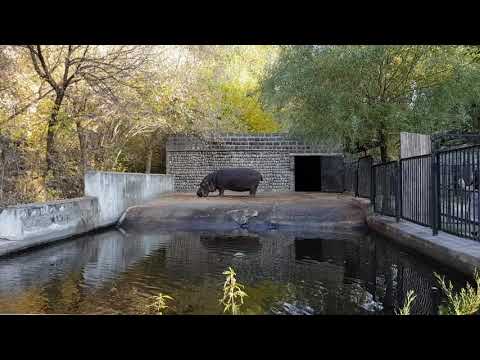This is a detailed photograph of a hippopotamus in its zoo enclosure. The image is framed by black bars at the top and bottom, emphasizing its horizontal rectangular shape. Centered in the photograph, the large hippopotamus stands on a gray asphalt-like surface, facing left with its nose close to the ground, as if sniffing. Behind the animal is a dark gray brick wall with a sloped opening on the right, possibly leading to its night shelter. To the immediate left is a low gray stone wall composed of two rectangular sections, with the one further in the background being taller.

On the right side of the picture is a tall black metal fence made of vertical bars. In the lower half of the photograph, there is a square-shaped pool of brownish water. The far background showcases a mix of trees: dense dark green foliage on the right, lighter green in the center, and bare-branched trees on the left. The foreground features sparse plant life, predominantly stems and weeds, adding to the natural outdoor ambiance of the scene.